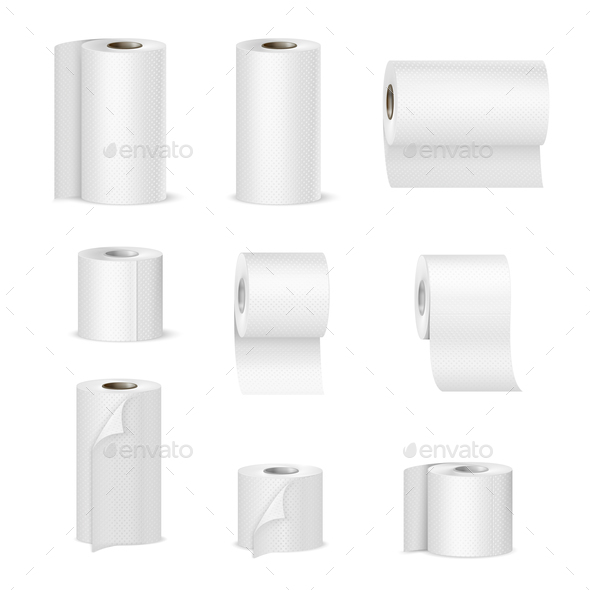This black-and-white image features nine rolls of paper products, divided into three rows of three images each. In the top row, we see three rolls of paper towels; the middle row showcases three toilet paper rolls. The bottom row consists of one paper towel roll on the left and two toilet paper rolls of different sizes on the right. The rolls are varying in size and orientation, all depicted in white or shades of gray, with gray-colored inner cylinders. The background is stark white with a watermark reading "Envato" in lowercase letters, placed in three locations across the image. The style is realistic, similar to what you'd find on a stock photo or digital imagery site.